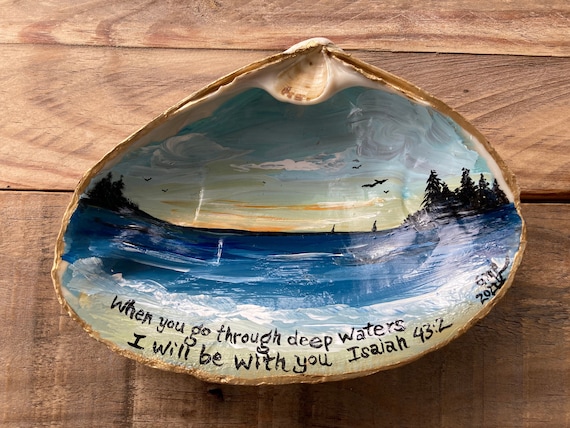This photograph captures a broken half of a large seashell, positioned upside down to reveal its inner surface. The seashell, resting on a wooden table with a natural or darker brown hue, has been beautifully decorated with a detailed painting. The painting depicts a serene sea scene, featuring a deep blue ocean that transitions to a lighter blue at the horizon to represent the sky. Above the horizon, the sky is light blue with streaks of yellow and green, hinting at sunset, while silhouettes of pine trees frame both sides of the shell, with five trees on the right and two on the left. 

Birds are seen flying across the sky, and streaks of sunlight illuminate the scene, adding to the tranquil atmosphere. At the bottom edge of the painted interior, a wave is depicted in white, adding a dynamic element to the ocean scene. Written on the wave in black lettering is the inspirational Bible quote, "When you go through deep waters, I will be with you," from Isaiah 43:2. The right edge of the shell features an artist's signature and the year "GRIP 2022," though the signature remains illegible. This evocative piece combines the natural beauty of the seashell with the thoughtful artistry of the painting, creating a striking visual and spiritual statement.